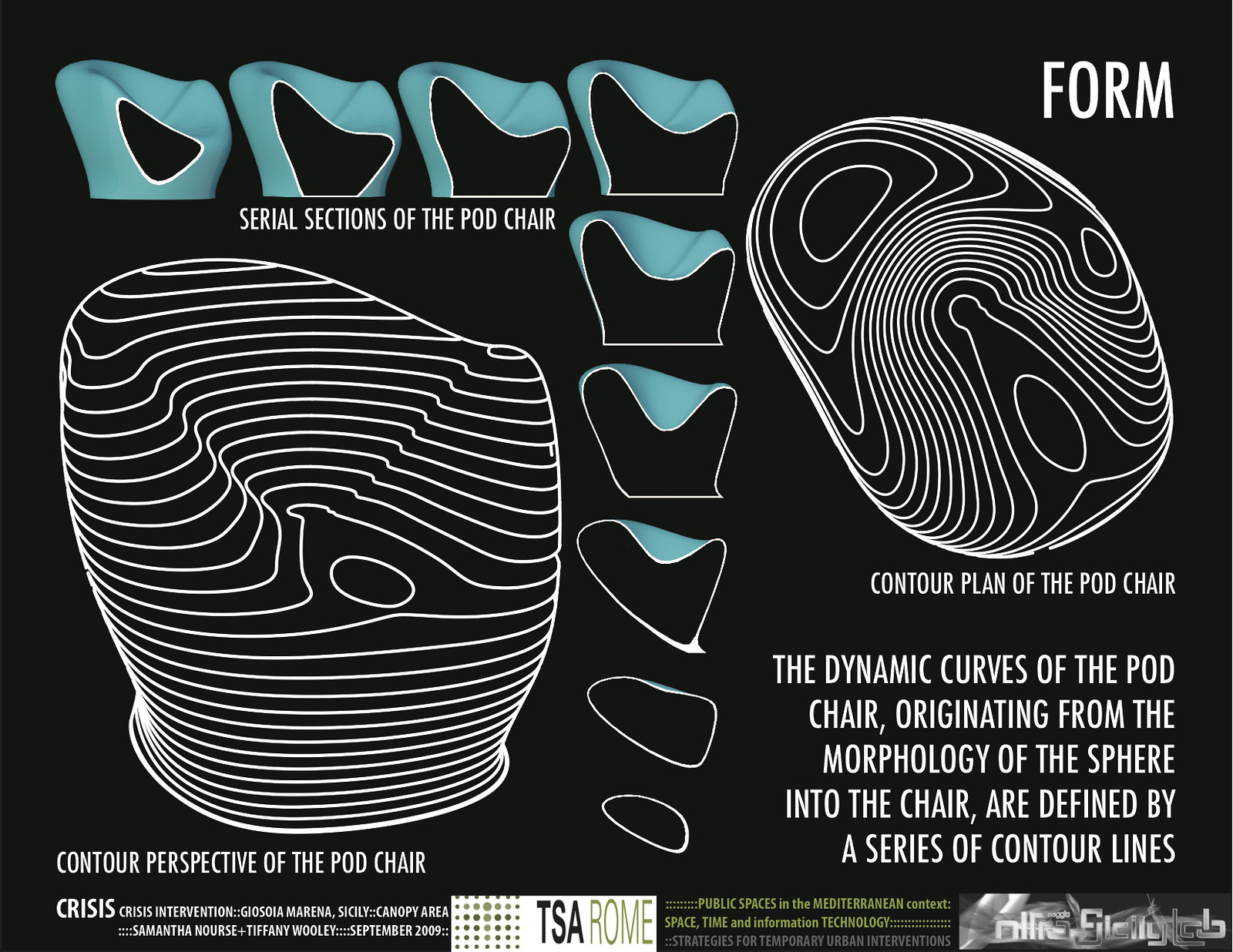This black-background poster advertises a contour pod chair, showcasing its ergonomic design and comfortable, orthopedic features. The primary visual elements include schematic sketches and dynamic illustrations detailing the chair's unique morphology from a spherical form to its final ergonomic shape. Notably, on the left side of the poster, there's a large black-and-white schematic demonstrating the interior construction of the chair, labeled "contour perspective of the pod chair." Adjacent to it, a series of blue illustrations in diminishing size traces the chair's evolution from top left to center, captioned "serial sections of the pod chair." In the upper right corner, large white letters spell "FORM," above a detailed contour plan. Further down, the text explains how "the dynamic curves of the pod chair originate from the morphology of the sphere into the chair, defined by a series of contour lines."

At the bottom of the poster, white lettering features names and details such as "Crisis, Crisis Intervention," "Geosuva Marena," and "Sicily Canopy Area." A white-on-black logo reading "TSA" is accompanied by lighter text stating "Rome." The lower right corner shows another logo, "OLLI Film Lab," in gray against a muddier background. Additionally, green text within the poster reads, "public spaces in the Mediterranean context, space, time and information technology, strategies for temporary urban intervention." The poster is dated "September 2009" and includes names such as "Samantha Norse" and "Stephanie Woolley."

Overall, the poster delivers a comprehensive overview of the contour pod chair's design, emphasizing its ergonomic qualities and the sophisticated process behind its creation.